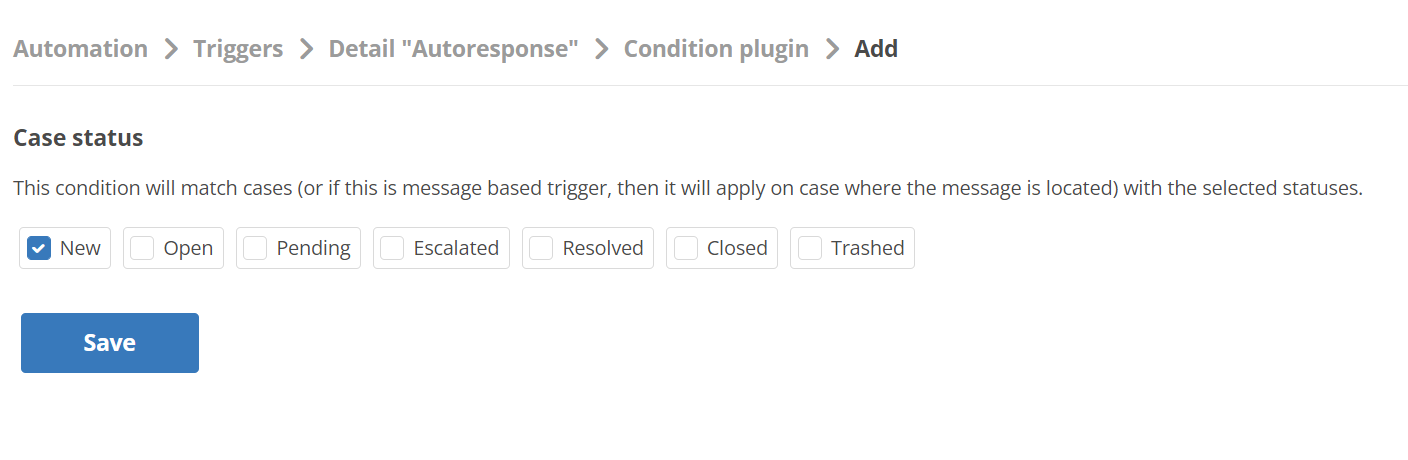Screenshot Description: 

The screenshot captures a desktop interface displaying a webpage that appears to be deep within the settings section of an application or website. The background is primarily white, with gray text prominently displayed at the top of the page. The section is titled "Automation" and features a series of options and settings related to triggers and conditional responses.

Key elements include:
- A subsection labeled "Detail Auto Response."
- A "Condition Plug-in" section which allows users to specify conditions under which certain actions will be triggered.
- Options to add new conditions or modify existing ones.

Below these headings, there is specific information regarding the "Case Status." Here, a description clarifies that the specified condition will match cases or, if it's a message-based trigger, it will apply to cases containing messages with the selected statuses. 

Accompanying this description are several checkboxes aligned horizontally, each representing different statuses:
- "New" (checked)
- "Open" (unchecked)
- "Pending" (unchecked)
- "Escalated" (unchecked)
- "Resolved" (unchecked)
- "Closed" (unchecked)
- "Trashed" (unchecked)

At the bottom of the page is a sizable blue button labeled "Save," intended to confirm any changes or additions made to the settings. The interface appears clean and straightforward, designed to help users manage automation and case statuses efficiently.